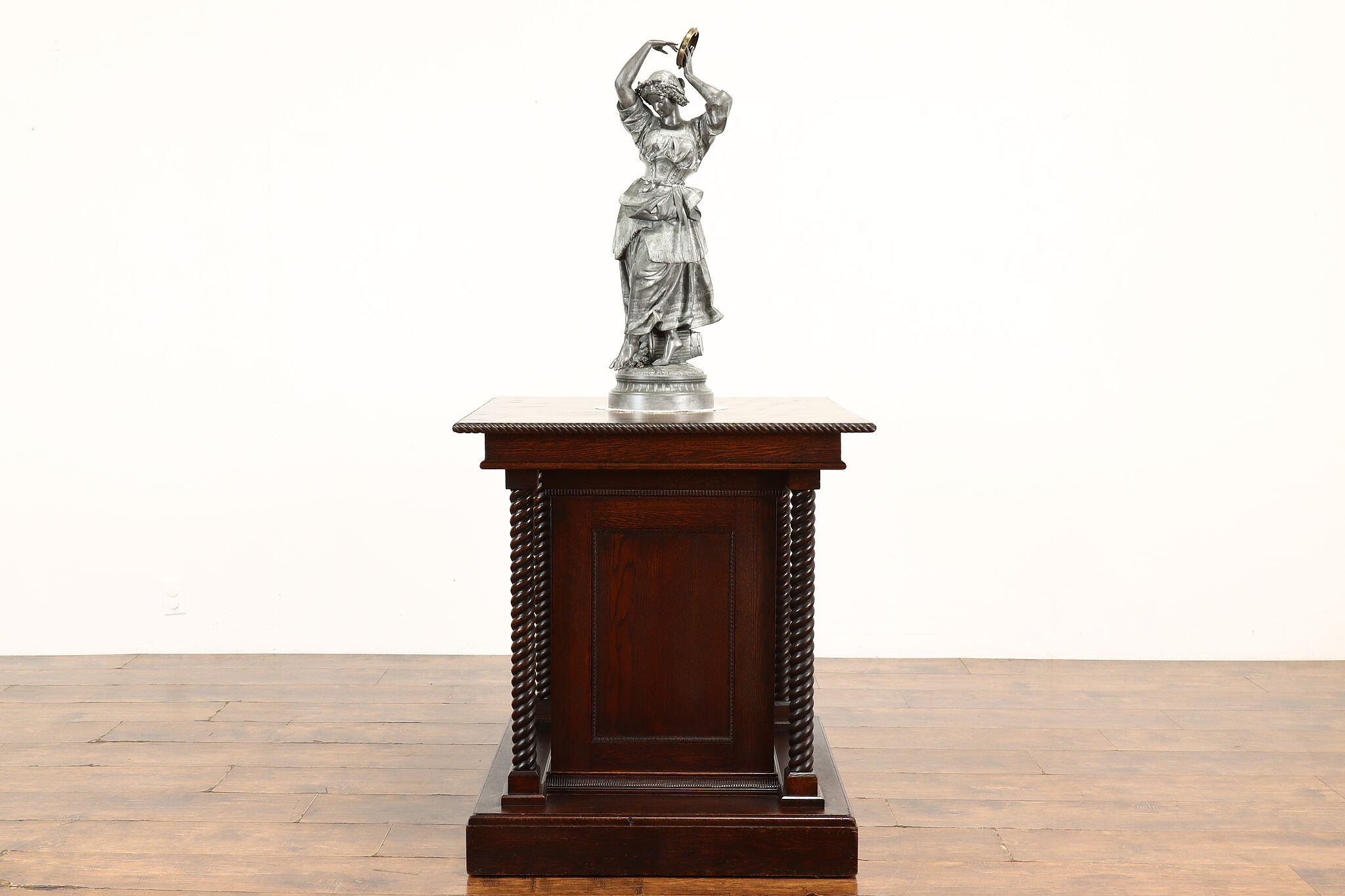This is a detailed photograph or illustration likely taken in an art gallery, showcasing a captivating sculpture. The artwork is prominently displayed on a substantial, dark wood base, which contrasts with the smaller scale of the sculpture, creating an interesting visual dynamic. The floor beneath the display stand is hardwood, enhancing the warm ambiance of the well-lit room, which features clean white walls. 

The sculpture itself depicts a woman in silver tones, captured in a dynamic pose that suggests she is dancing or performing. She is dressed in a flowing long dress with voluminous sleeves and appears to have a wrap around her waist, adding layers to her skirt. Her arms are elegantly raised above her head, and she is holding a tambourine in her left hand, tapping it with her right, while also wearing a turban-like headpiece. Although the sculpture is small and detailed features are hard to discern from a distance, its shiny metallic surface highlights its intricate craftsmanship. The woman stands on a metal pedestal that is harmoniously set atop the wooden display base, creating a striking composition that captivates the viewer's attention.